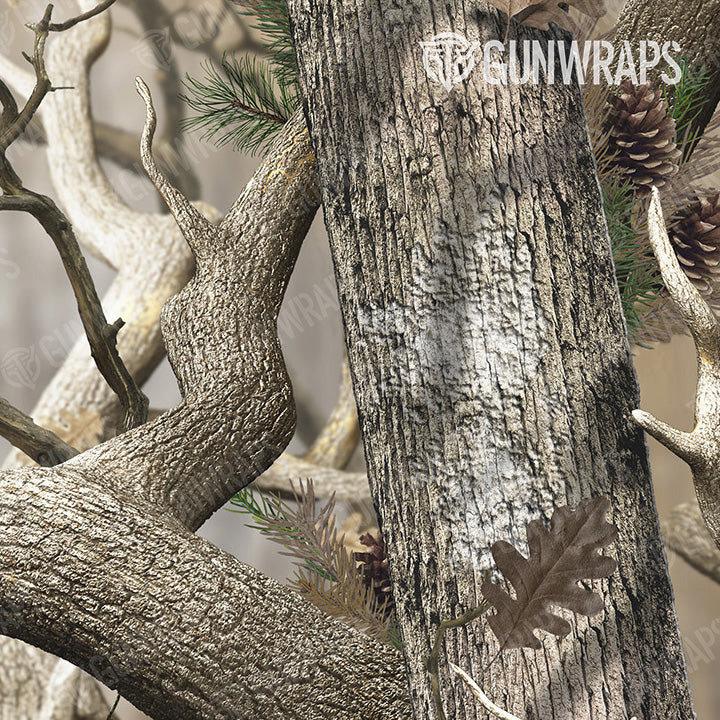This is an intricate color photograph, or potentially an AI-generated image, that mimics an abstract piece of art featuring a loosely layered arrangement of various tree branches and pieces of wood. The elements range in a white to brown color palette, dominated by beige and tan hues. Some branches appear intertwined, wiggling together in a natural composition with occasional white staining, evoking a serene autumn atmosphere. 

You can spot green pine leaves and multiple pine cones scattered throughout the scene, along with brown leaves—one of which is prominently stamped against a main tree trunk. The branches possess a classic tree trunk appearance varying in shades, with some light enough to almost resemble antlers. Occasional pieces of green fern add a touch of verdant contrast amidst the fall colors.

A subtle shadow casts onto the blank space behind the arrangement, enhancing its depth. The photograph is marked by a barely noticeable, transparent watermark with "Gunwraps" running lightly across the image. Additionally, the top right corner of the photograph prominently displays the "GUNWRAPS" logo in uppercase white lettering, accompanied by a small emblem positioned to the left of the 'G'.